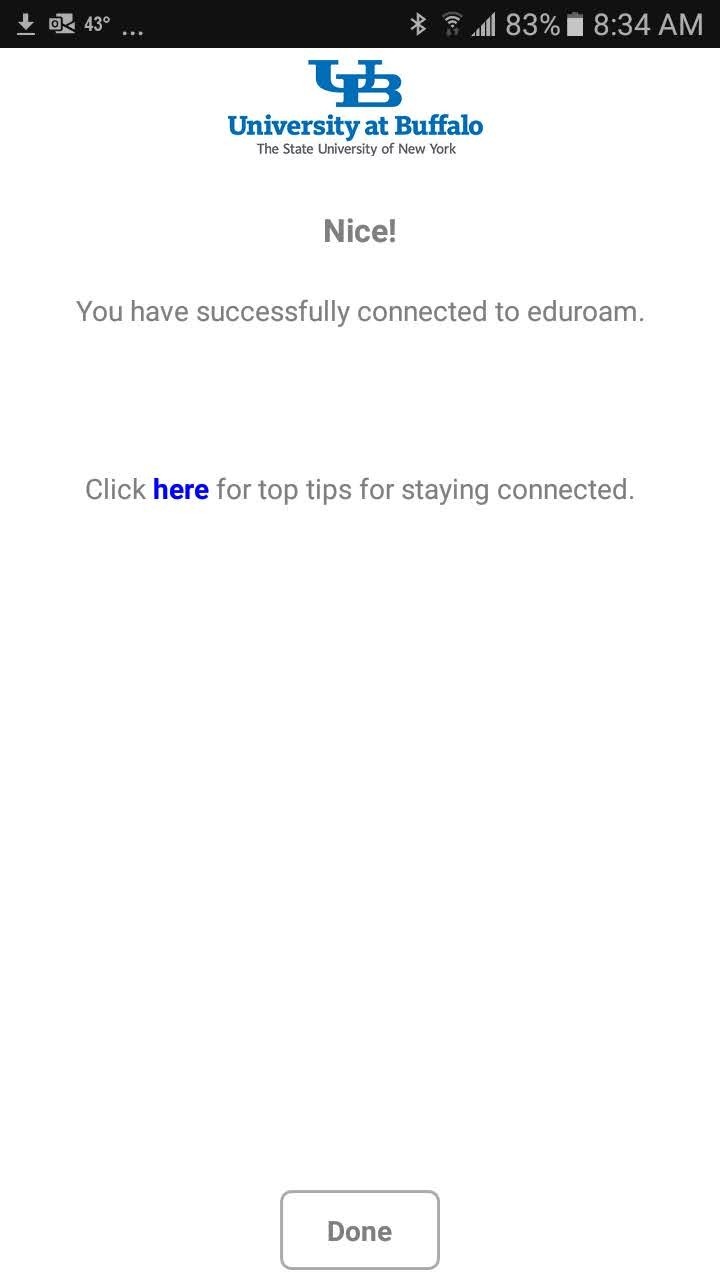The image is a screenshot taken from a mobile phone. In the upper left corner, there are a few symbols: a download icon, an unidentified symbol in the middle, and '43°'. On the right side of the screen, various status indicators appear, including Bluetooth, mobile service bars, and a battery icon displaying 83% charge, along with the time '8:34 AM'.

Below these status icons, 'U' with a 'B' over it is displayed in blue text, followed by 'University at Buffalo'. In smaller, black text beneath this, it reads 'The State University of New York'. Centrally positioned on the page, the text 'NICE!' is prominently displayed, followed by the message, 'You have successfully connected to eDuro AM. Click here for top tips for staying connected.' The phrase 'Click here' is in hyperlink blue text, indicating it's a clickable link. 

The rest of the screen exhibits a significant amount of white space. At the very bottom center, there is a 'DONE' button, which is outlined in black with the text in black as well on a white background. The phone's specification icons and text are displayed with a contrasting black background with white text.